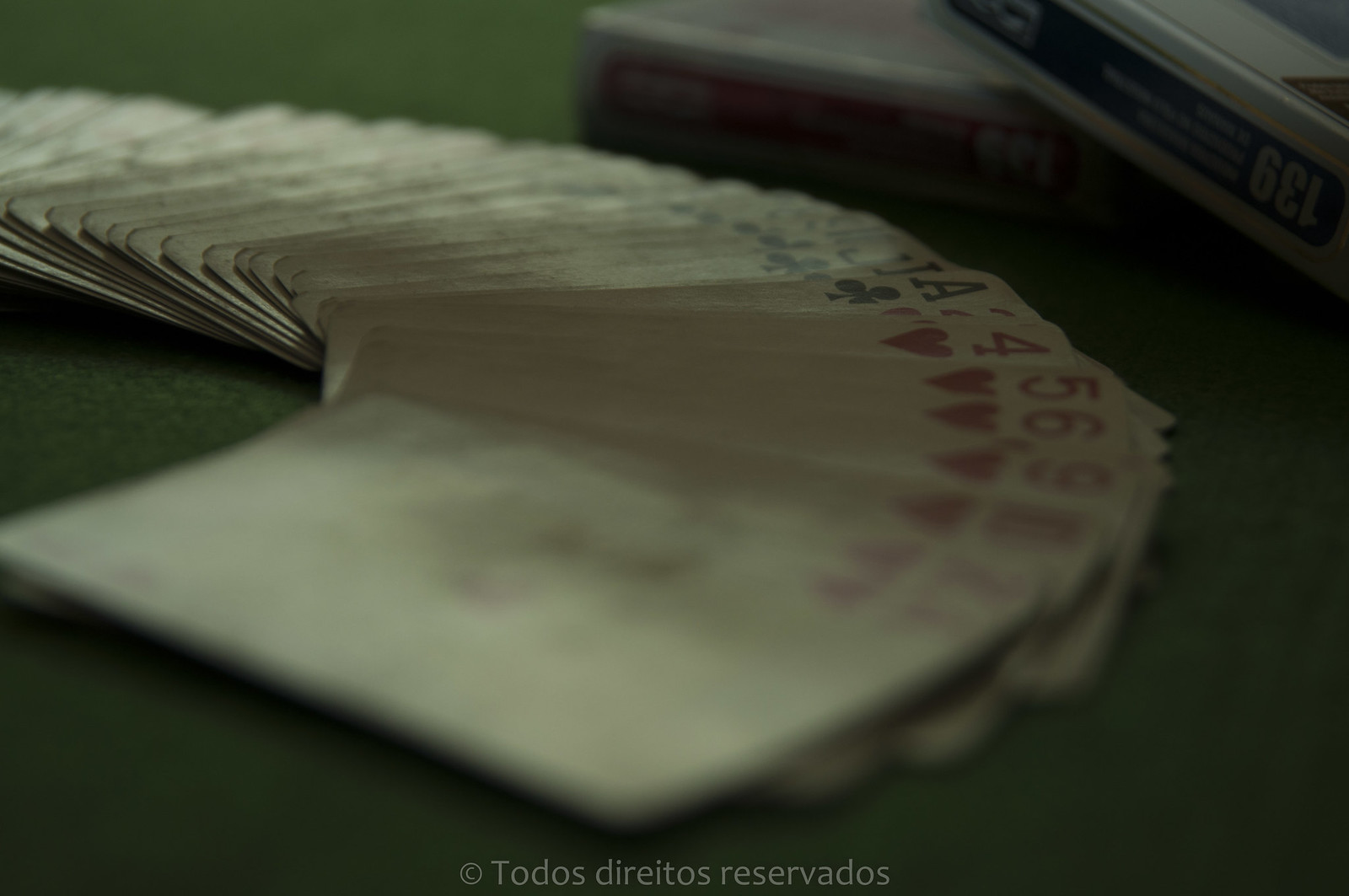The image portrays a dimly lit scene featuring a stack of playing cards arranged in an elegant, arched pattern reminiscent of a dealer's spread at a casino. The cards are stacked in such a way that each one slightly overlaps the other, cascading to the right. Despite the darkness of the background and the cards themselves, there is a faint light that reveals their presence, although no specific details such as faces or lettering are discernible. The somber tones dominate the image, rendering it almost monochromatic with a black background. At the bottom of the image, there is text that reads "TOTOS, DORITOS, RESERVADOS," adding a cryptic element to the scene. The total number of cards is estimated to be around fifty.